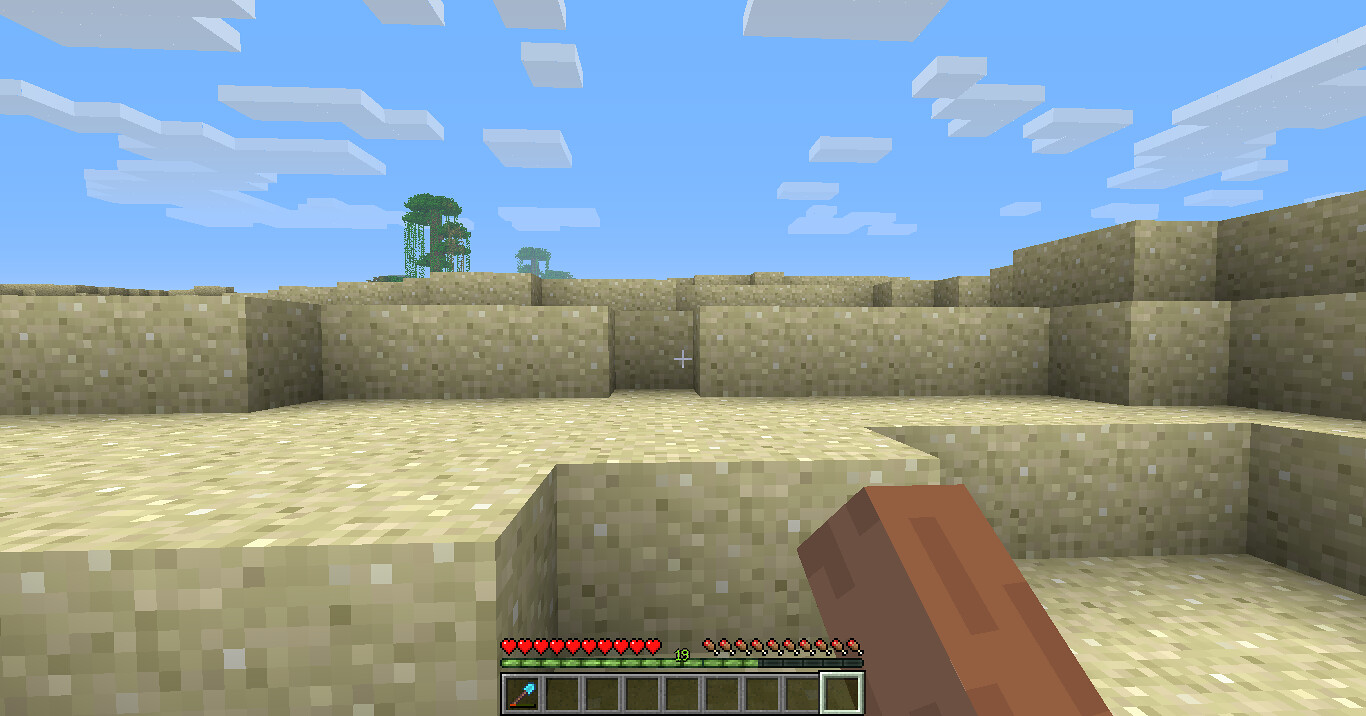The image depicts a pixelated, block-style screenshot from a computer game, reminiscent of Minecraft. The sky overhead is a soft blue, scattered with square and rectangular white and grey clouds. The landscape is composed of greenish-brown blocks arranged at varying heights, creating a stepped terrain that the character can navigate. In the distance, pixelated green trees with brown trunks can be seen, adding depth to the scene. In the foreground, on the right side, there is an angled wooden block or post, resembling a gun or a stick. Centered at the bottom of the screen is a game interface with grey squares, icons, and a scoring legend. Visible are several hearts, a green energy bar marked with the number 19, and an icon for a spade. A small cross is positioned in the center of the image, enhancing the sense of focus within the game.